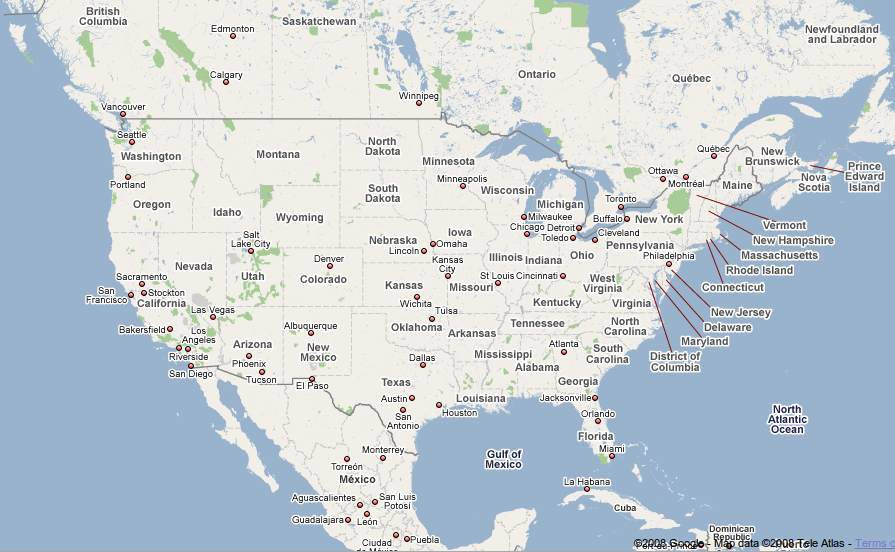This digital creation is an intricately detailed map of the United States, extending to include portions of Mexico and Canada. Effectively presenting a broader representation of North America, the map omits the often included inset of Alaska and Hawaii but spans extensively from British Columbia to Newfoundland in Canada. Every U.S. state is depicted, except Alaska and Hawaii, alongside comprehensive labels identifying state capitals. A significant part of Mexico is also charted, along with select capitals, and Cuba is notably included. The map meticulously labels major bodies of water such as the Gulf of Mexico and the North Atlantic Ocean. Canadian cities like Calgary and Edmonton in Alberta, Vancouver in British Columbia, Winnipeg in Manitoba, and Quebec City in Quebec are marked, while certain regions like Saskatchewan and Newfoundland have no cities listed.